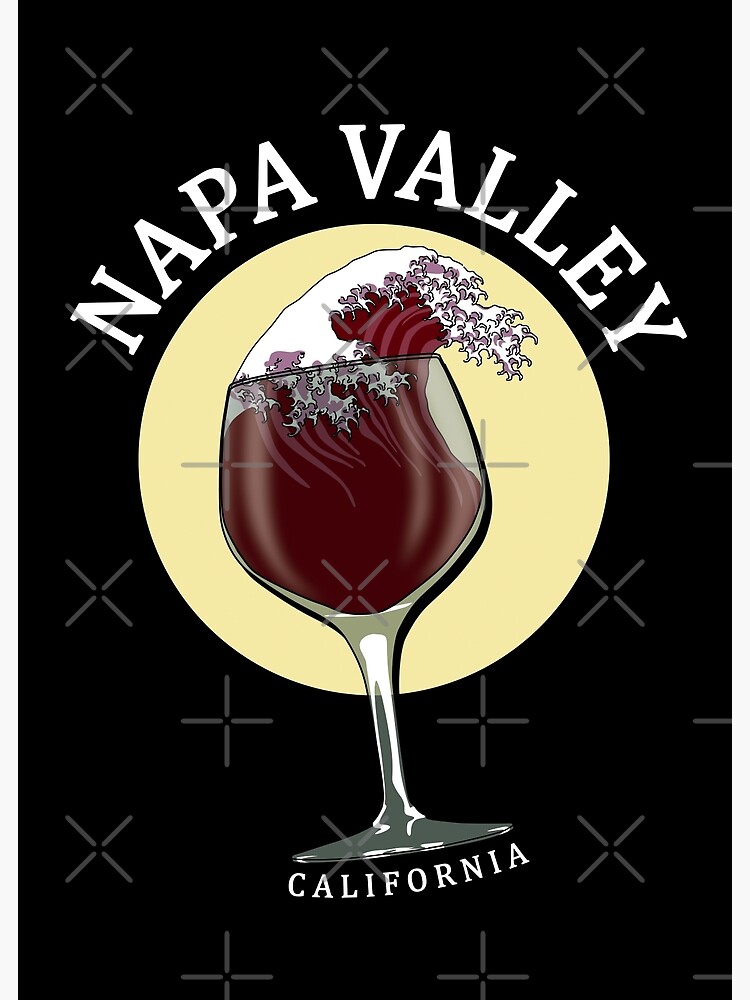The image is a computer-generated piece of art with a predominantly black background, featuring numerous grey X's scattered throughout, possibly as watermarks or for copyright protection. Across the top of the image, in large white capital letters, it reads "NAPA VALLEY." Central to the image is a tall wine glass, from which the wine appears to foam over in the style reminiscent of traditional Japanese wave art, characterized by specific line patterns and shading. Behind the wine glass, there's a pale yellow circle, evoking the impression of the sun. At the very bottom of the image, beneath the glass, the word "CALIFORNIA" is written in white capital letters, though in a slightly thinner font compared to the text at the top.